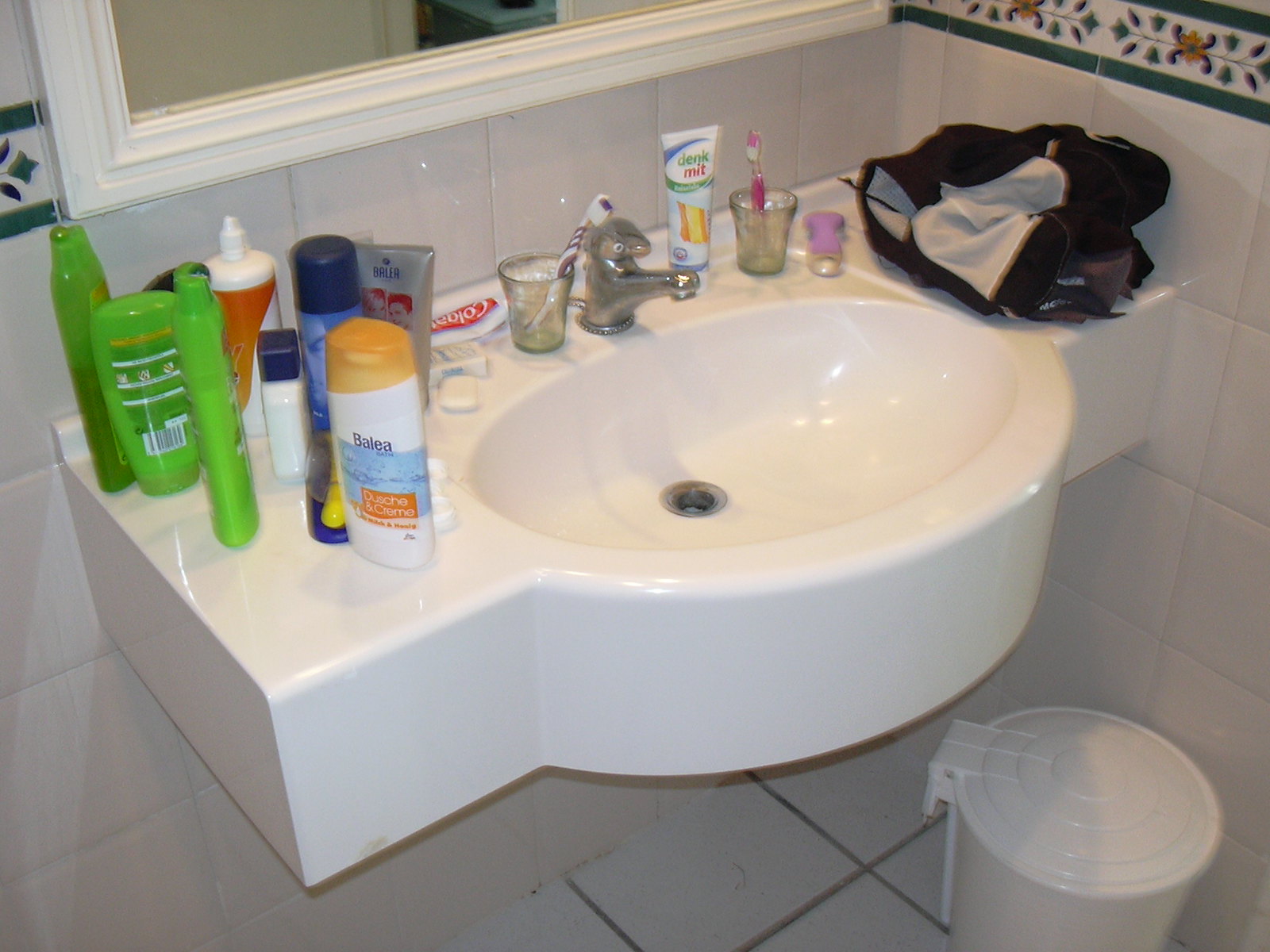This photograph captures the details of a household bathroom. The focal point is a white, wall-mounted countertop with an integrated oval sink, which slightly protrudes from its front edge. To the right of the sink, a black garment with a white lining is draped, accompanied by a cup holding a pink toothbrush and a tube that appears to be toothpaste, although the text on it is not in English. On the left side, another cup containing a purple and white toothbrush sits next to an unwrapped bar of soap and a tube of Colgate toothpaste. The left side of the sink also features an array of green shampoo and conditioner bottles, along with various other health and beauty products. The room's aesthetic consists of a white tile floor with dark grout and white tile walls with white grout. A decorative floral border in green, white, and pink or peach hues adorns the top portion of the wall, above which a white-framed mirror is precisely aligned with the border's bottom edge. Nestled partially beneath the sink is a small white plastic garbage pail with a hinged lid.